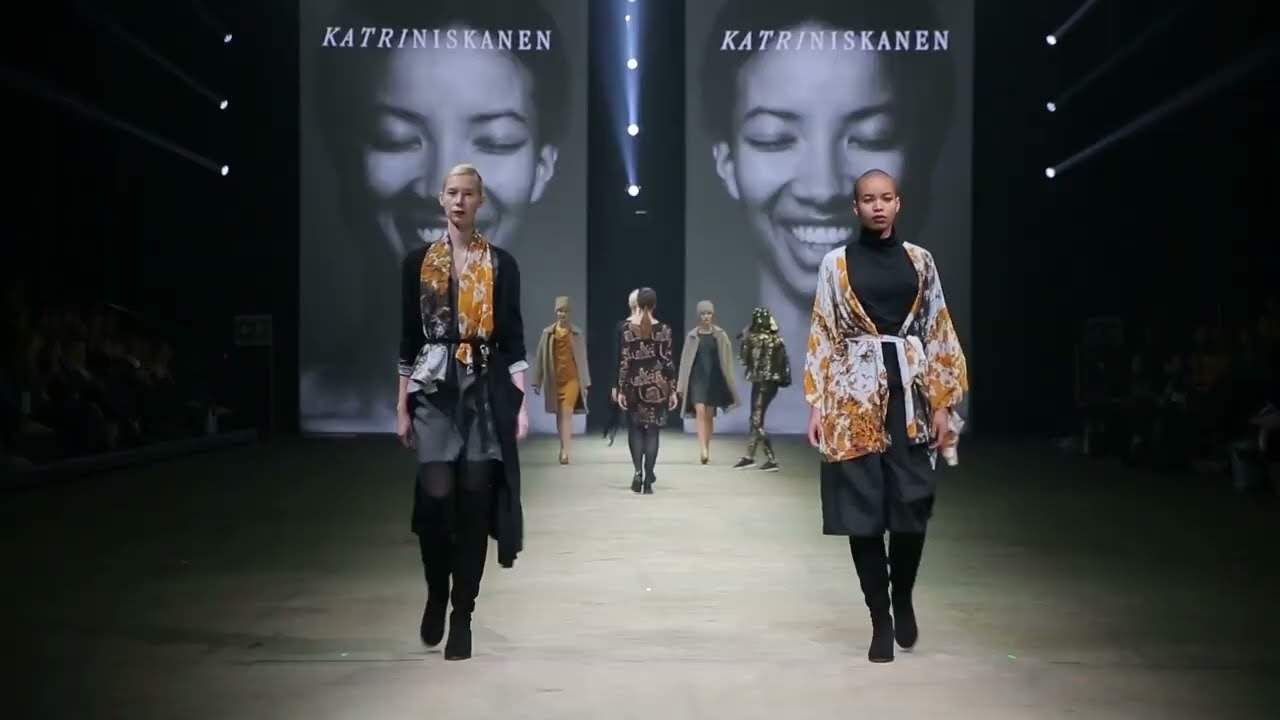The image captures a vibrant scene from a fashion show set in a spacious, industrial-like room with cement floors and minimalistic decor. The audience is seated in darkened areas at the edges of the image, creating a stark contrast with the brightly lit center where the models are walking. In the background, large vertical billboards display a close-up photograph of a smiling woman with her eyes closed, overlaid with the name "Katrinis Kanin" in white text.

Dominating the foreground, two models walk towards the viewer. On the left is a tall, thin blonde with short hair, wearing a striking ensemble consisting of a yellow-white and black scarf draped over a black cropped jacket, paired with a silver and black dress and black boots. To her right is another model with a shaved head and a more robust build. She sports a black dress and black boots underneath a distinctively colored small kimono, featuring hues of white, yellow, golden-yellow, and black.

Both outfits cleverly play with dark tones, accentuated with splashes of color and standout pieces such as the scarves and kimonos, creating an eye-catching contrast that aligns with the show's bold aesthetic. The models’ confident strides and the eclectic, fashionable designs suggest a theme of modern elegance infused with a touch of industrial edge, perfectly captured in this thrilling moment from the fashion event.